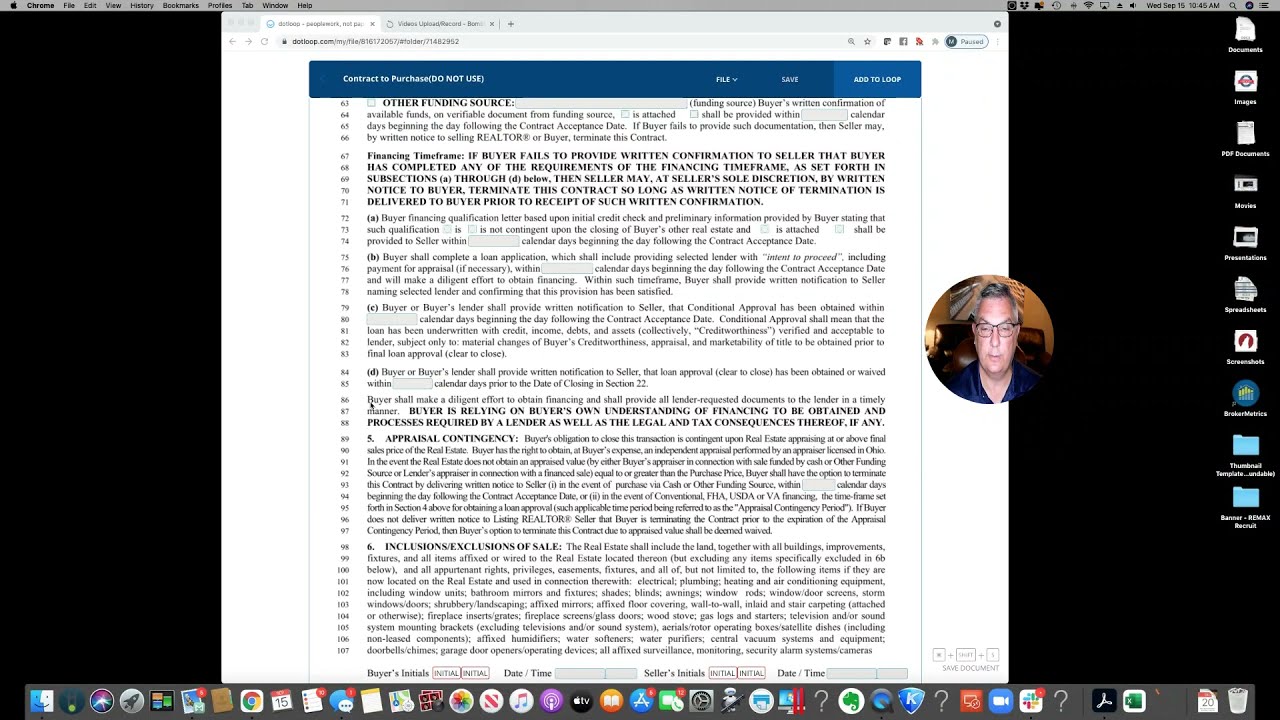The image is a detailed screenshot of a man's computer screen during a Zoom video call. Predominantly, it showcases a white Microsoft Word document, centrally situated, with several paragraphs of black text, including bolded and numbered lines, rendered atop a contrasting black background. This Word document has a blue header that seems to suggest it might be a purchasing document with phrases like "connect to purchase," and "do not use." 

The bottom of the screen features the distinctive logo and menu bar of an Apple Macintosh computer, populated with a variety of QuickLink applications. Similarly, a vertical array of icons for different files and applications runs along both the left and right edges of the screen. These are set against the plain black desktop background.

Overlaying the document, on the right-hand side, is a circular Skype-like window showing a close-up of an older Caucasian man, likely in his 50s or 60s, wearing glasses. His video feed suggests he is in his living room.